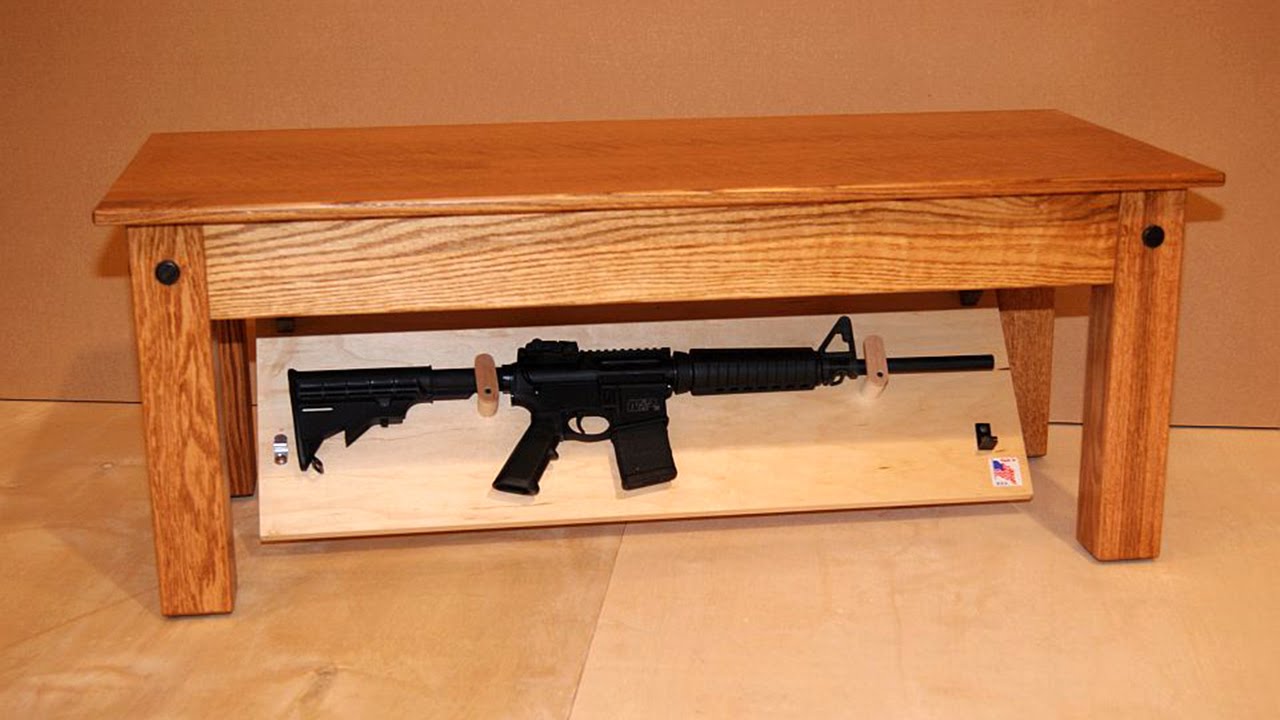The photograph features an intricately detailed setup centered around a large black assault rifle displayed on a wooden placard. The rifle, secured by metal brackets and wood holders, has a notably long barrel and chamber, suggesting it’s a significant firearm, possibly of military origin. This placard, bearing a prominent American flag sticker on the lower right-hand side, hints at a patriotic or military display. The entire setup is intriguingly placed underneath a light brown wooden coffee table, which is rectangular and simple in design, featuring visible black screws. The background of the setting includes a brown wooden wall and a two-toned brown tile floor, adding to the rustic and solemn ambiance of the room.